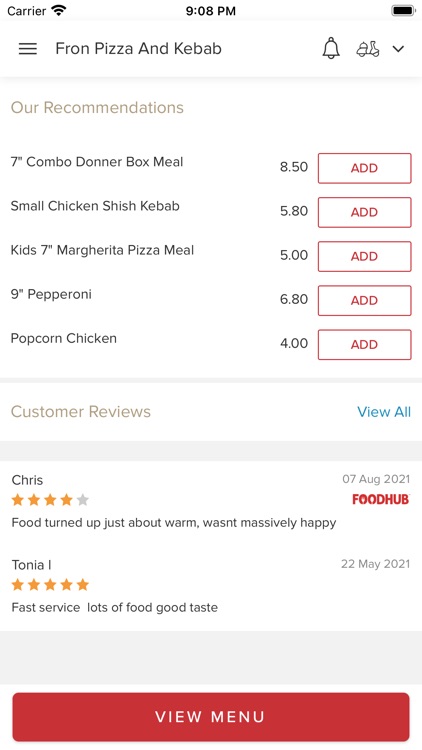This is a detailed screenshot from a cell phone, captured in portrait orientation, featuring a mobile app interface for a restaurant named "Fran Pizza and Kebab." The image lacks a defined border and is considerably taller than it is wide, mimicking the proportions of a cell phone screen.

At the very top left, the word "Carrier" is displayed, indicating the cell service provider, followed by an almost full Wi-Fi signal icon. In the center of the header, the current time is shown as "9:08 PM" in black font. Adjacent to this, on the far right, there is a horizontal battery icon that is nearly full.

Directly below the header, there is a sub-header with a hamburger menu icon on the left. Beside it, the name of the restaurant "Fran Pizza and Kebab" is prominently displayed. To the right of the name, there are several icons including a notification symbol, a moped icon likely indicating delivery options, and a downward arrow suggesting additional menu options.

Following this sub-header, there is a grey-font section titled "Our Recommendations" presented within a distinct rectangular box. This section lists five menu items with prices: $8.50, $5.80, $5.00, $6.80, and $4.00. Each price has an accompanying red rectangle labeled "Ad."

Below the recommendations, there is another section for customer engagement, featuring a grey-font title within a white box that reads "Customer Reviews" followed by a "View All" option.

Further down, two individual customer review sections are visible. The first review is from a user named Chris who has rated the restaurant four stars. The second review comes from Tanya, who has given the establishment a five-star rating.

Overall, the screenshot showcases the Fran Pizza and Kebab mobile app interface, providing users with menu recommendations and access to customer reviews, set against a primarily white background with minimalistic design elements.